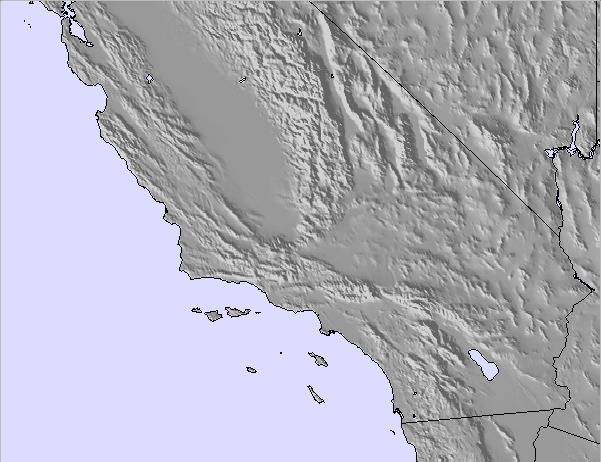The image is a landscape-oriented, color-illustrated map focusing on a continent-like landmass that is predominantly gray, suggesting rocky terrain. The landmass is intricately detailed with features such as mountains and various small islands off its western coast. Unique characteristics include a light purple, lavender-hued ocean bordering the land, and the addition of green highlights, most prominently towards the top of the map, which may signify elevated terrain or vegetation. Black stripes delineate different territories, adding a layer of complexity to the geography. Additionally, a small, similarly light purple body of water is located at the map's corner, perhaps indicating a lake or a sea. The map appears inverted and includes various lakes within the state, the largest of which is shown in the same light purple shade as the coastal waters. The detailed cartographic style and vivid color choices enhance the map's textured and illustrative quality.